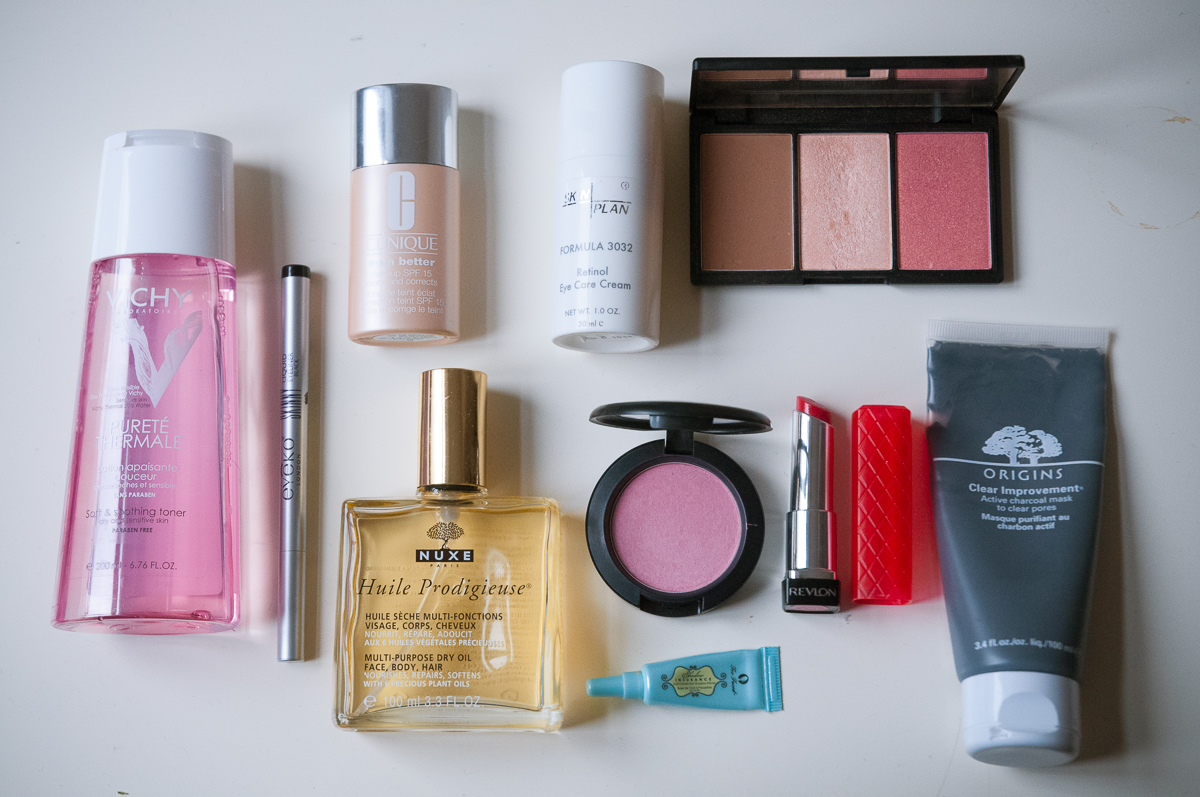The image depicts an assorted spread of a female makeup kit meticulously arranged on a pristine white background. 

On the left side of the arrangement, a pinkish perfume bottle catches the eye with its delicate hue. Centrally positioned is a sleek bottle of Huy Prado Juice by Huy Ngoc, suggesting an aromatic perfume. Just beside it, a gray container of Origins Clear Improvements, presumably housing a luxurious cream or shampoo, stands in contrast.

Nearby, a small blue container and an elegant red lipstick lie in tandem, the latter with its casing slightly ajar, revealing the vibrant lipstick inside. Adjacent to these is a pink mascara accompanied by an open mirror, hinting at its practical application.

A Clinique bottle filled with tan liquid or cream adds to the array of high-end cosmetics. Further along, a white bottle labeled Plan Formula 3022 Eye Care Cream stands out, promising specialized skincare.

Completing the ensemble is a sophisticated compact of skin powder, displaying a spectrum of complementary shades from tan and beige to a warm reddish hue, paired with a mirror propped up for convenience. Lastly, a subtle inclusion of a pen, identifiable as a Siggrove pen, is also part of the assortment, though its details remain partially obscured.